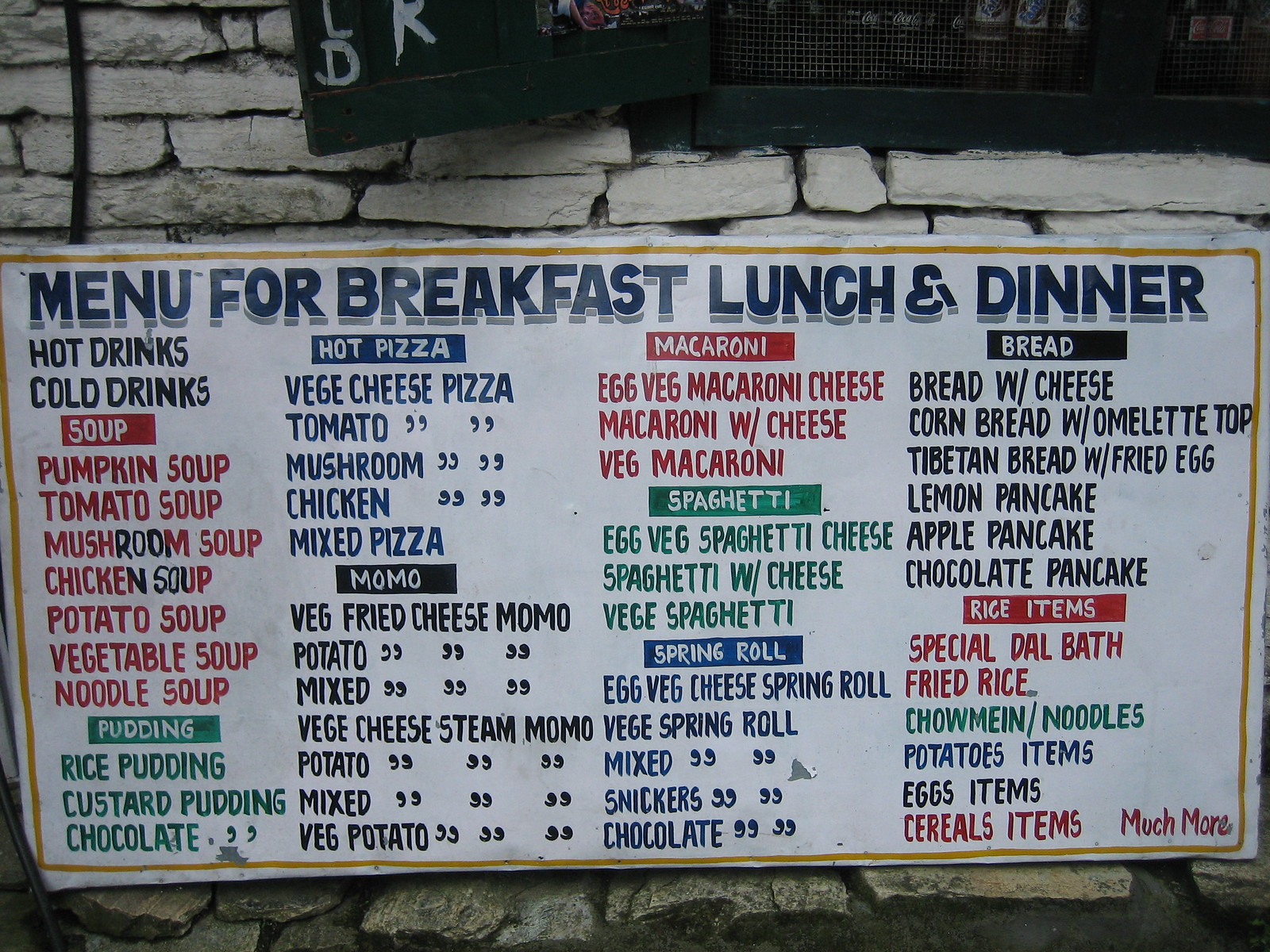The image depicts an extensive menu displayed on a textured cobblestone wall. The menu comprehensively lists a variety of food and drink items available for breakfast, lunch, and dinner, arranged in several columns with colorful headers.

In the first column, the "Hot Drinks" and "Cold Drinks" sections top the list, followed by a variety of soups—pumpkin, tomato, mushroom, chicken, potato, vegetable, and noodle—all written in red. Beneath this section, a green rectangle labeled "Pudding" lists different puddings: rice pudding, custard pudding, and chocolate pudding.

The second column features a blue rectangle titled "Hot Pizza," with options such as veggie, cheese pizza, tomato pizza, mushroom pizza, chicken pizza, and mixed pizza all written in blue. Below that, the section labeled "Momo" offers various momo options: veg fried cheese momo, potato fried cheese momo, mixed fried cheese momo, veggie cheese steamed momo, potato cheese steamed momo, mixed cheese steamed momo, and veg potato steamed momo, all written in black.

In the next column, a red header introduces "Macaroni in a Box," featuring egg, veg, macaroni, cheese macaroni, macaroni with cheese, and veg macaroni, all written in red. Underneath, a green box titled "Spaghetti" lists egg, veg, spaghetti, cheese, spaghetti with cheese, and veggie spaghetti—all written in green. Below this section, a blue rectangle denotes "Spring Roll" offerings, including egg, veg, veggie, mixed, Snickers spring roll, and chocolate spring roll, all listed in blue.

The final column, with a black box titled "Bread," offers selections such as bread with cheese, cornbread with omelet top, Tibetan bread with fried egg, lemon pancake, apple pancake, and chocolate pancake. This column also includes a section called "Rice Items," listing a special dhal bath fried rice. Below that, in green ink, it features "Chow Mein / Noodles," followed by "Potato Items" in blue, "Egg Items" in black, "Cereal Items" in red, and concludes with "Much More."

The vibrant colors and varied sections make the menu both appealing and comprehensive, catering to diverse tastes and dietary preferences.